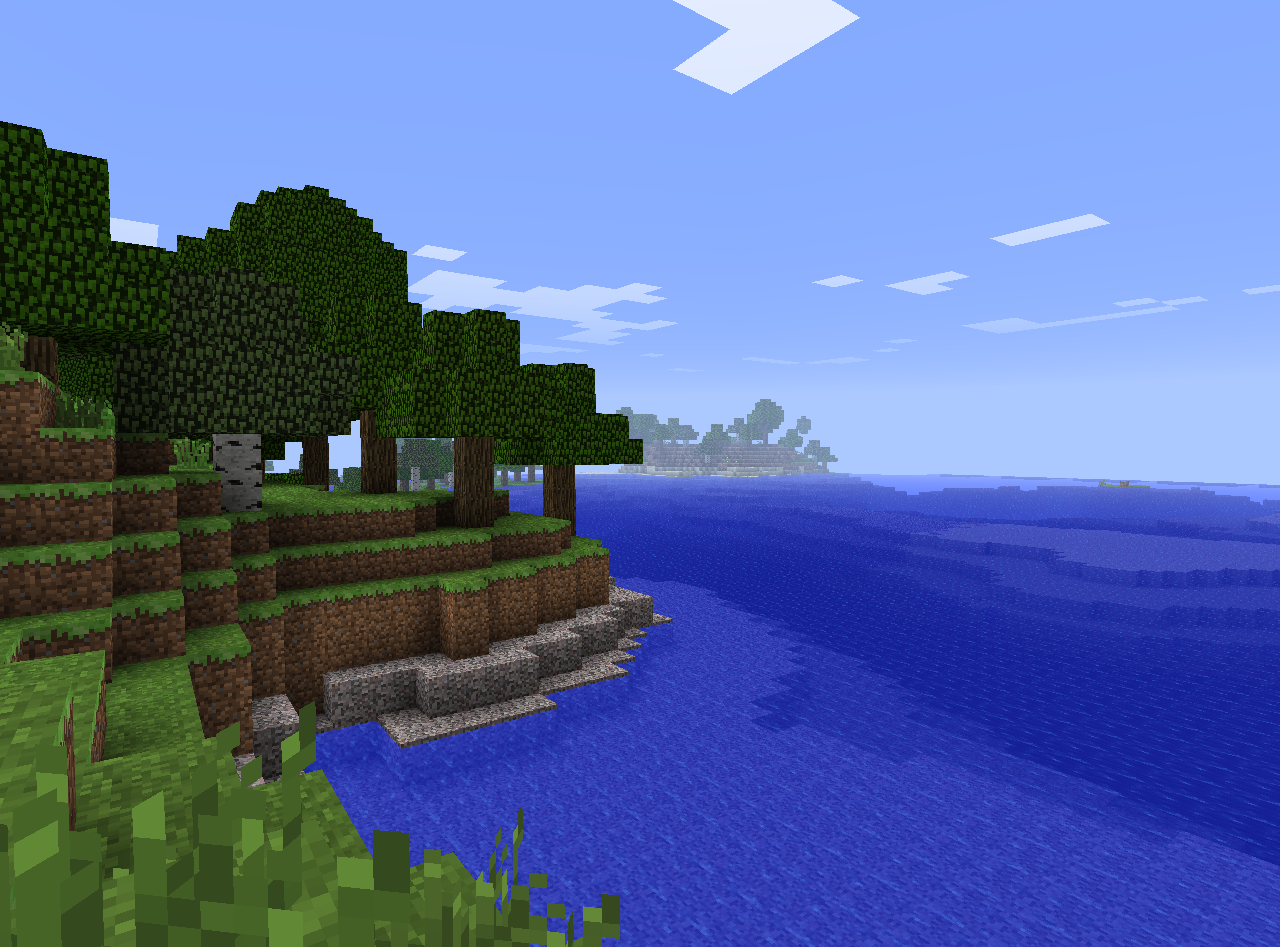A picturesque still image from a Minecraft game captures the tranquil juncture where ocean meets land. On the right side of the image, stretching into the middle, the ocean enthralls with its dark blue waters that gradually lighten as they extend towards the horizon. The left side showcases the vibrant landscape, featuring lush green grass that gently staggers and tapers down to the water's edge. Atop the land stand an array of trees, some adorned with lighter green foliage while others boast darker green leaves, all supported by trunks varying from deep to light brown. In the distance, an island emerges, rising in a gentle hill shape and dotted with multiple trees, adding depth to the scene. The sky above is a serene expanse of blue, adorned with a few wisps of white clouds that also lighten as they near the ocean.